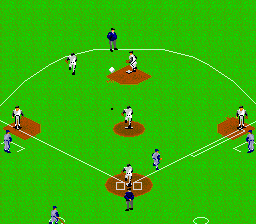This image appears to be a screenshot from an old Nintendo-era video game, presenting a baseball field in an 8-bit graphic style. The image is relatively square in shape and features a textured green background, simulating grass. White lines outline the baseball field, clearly defining the bases and boundaries. The bases, which are brownish with cut-off corners and reddish outlines, include a circular home base with two white rectangles and a reddish border, likely depicting the batter's box.

In the foreground, a player in a blue shirt, gray pants, and dark shoes stands behind home plate. This player appears distinct from the others. The team currently fielding is wearing white uniforms, complemented by dark caps, sleeves, and shoes. Their opponents, the batting team, are donned in gray uniforms with dark blue shirts and dark shoes.

The gameplay is captured with players positioned strategically: the white-clad defenders cover the field while a member of the gray team runs from home base toward first base. Another gray player stands near first base. Additionally, a figure in a dark blue shirt and gray pants, presumably a referee, stands behind second base to oversee the action. Another defender in white is situated between second and third base, along with white-clad players guarding each base. Moreover, a gray batter can be seen in the bottom left corner of the image, ready for their turn.

The scene effectively encapsulates the nostalgic feel of early video game sports simulations, down to the pixelated aesthetic and simplified player animations.